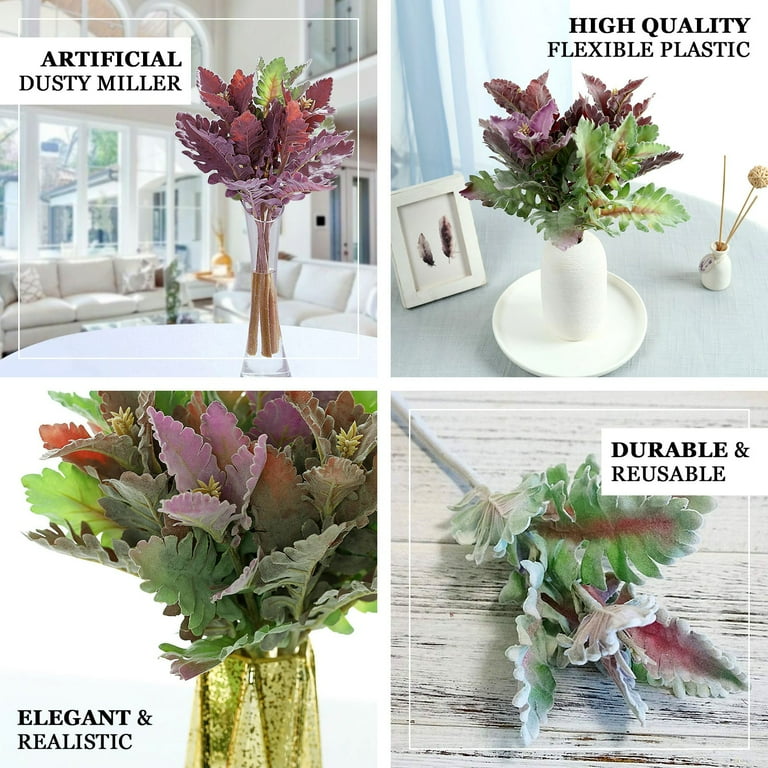This image collage advertises artificial Dusty Miller plants through four detailed panels. The upper left panel displays a collection of these plants in a tall, clear, white vase filled with water set against a bright, beige living room backdrop featuring ample natural light streaming through large windows. The upper right panel showcases the plants in a white, stocky vase on a saucer, placed on a round table draped in a light gray tablecloth, with a photograph resembling insect wings and soft light blue walls in the background. The lower left panel offers a close-up of the faux plants in an elegant gold-toned glass vase, highlighting the lifelike blend of green, maroon, and red foliage, labeled "elegant and realistic." The lower right panel emphasizes the product's durability, describing the artificial plant as "durable and reusable," with the plant shown against a rustic, whitewashed wooden surface.